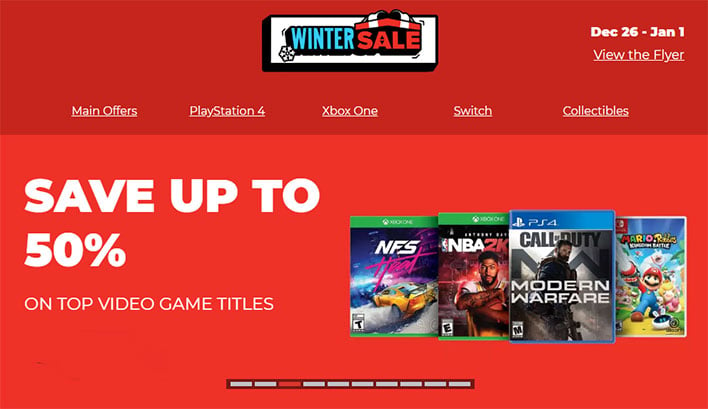**Winter Sale Announcement for Gamers**

*Website Layout:*
The webpage is predominantly red, with a darker red top bar and a lighter red bottom bar. 

*Header:*
At the top center of the page, enclosed in a white, black-bordered rectangular box, is the announcement "Winter Sale." The word "Winter" is in an aqua font outlined by black, while "Sale" is in a red font outlined by black. Positioned above the text is the top portion of a gift box. A snowflake icon decorates the lower-left corner of the word "Winter." 

*Event Dates:*
In the upper right corner, the dates "Dec 26th - Jan 1st" are displayed in white font. Beneath these dates, there is a clickable link labeled "View the flyer."

*Navigation Bar:*
The dark red top bar contains five headline links: "Main Offers," "PlayStation 4," "Xbox One," "Switch," and "Collectibles."

*Main Content:*
Beneath the navigation bar, large white text reads "Save up to 50%," followed by a smaller caption specifying "on top video game titles."

*Featured Video Games:*
To the right of the page are images of four video games:
1. **NFS Heat (Xbox)**
   - Cover Image: Depicts a yellow race car.
   - Design: Green banner at the top, white font with "Heat" in pink.
2. **NBA 2K**
   - Cover Image: Features an African American basketball player with black hair, a beard, a mustache, and tattooed arms crossed.
   - Text: "NBA" in white, "2K" in red.
3. **Call of Duty: Modern Warfare (PS4)**
   - Cover Image: Displays a soldier.
   - Text: "Call of Duty" in black, "Modern Warfare" in white.
4. **Mario Brothers**
   - Cover Image: Showcases Mario holding a white laser gun, with two characters behind him.
   - Design: Mario wears a red hat, black mustache, and blue overalls with a red shirt.

*Footer:*
At the bottom of the page, navigation controls indicate that the user is on the third page with a total of ten pages available for browsing.